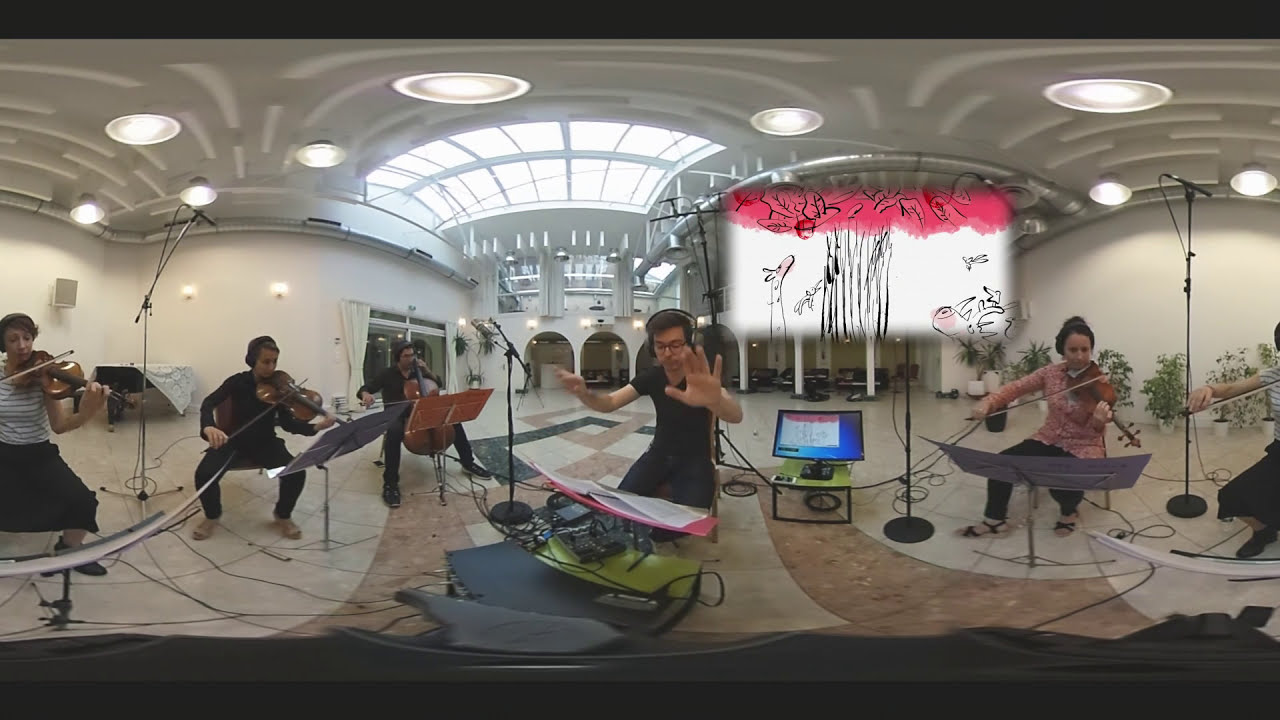This photographic image captures an indoor musical performance within a spacious, well-lit concert hall. The scene is taken with a wide-angle lens, causing the entire setting and participants to appear slightly curved. Centered prominently in the composition is a male conductor, who is seated, wearing headphones, glasses, and a black shirt, with his hands animatedly guiding the musicians. Around him are five violinists—three women and two men—seated on black chairs, clad in various outfits. A woman in a gray striped shirt and another in a pink shirt with black pants and sandals are among the female violinists. The men include one wearing all black, playing a cello, and another man also in black playing a violin.

Microphones on stands are strategically placed near the instruments, capturing the intricate sounds of the performance. In the background, a large screen displays a graphic showing a tree with pink leaves, a black trunk, a giraffe on the left, and a rhinoceros on the right, creating an immersive backdrop. Beneath the screen, there appears to be a computer and additional microphone stands. The surroundings feature a tan and brown colored floor, bright recessed lighting on the gray ceiling, and a skylight illuminating the room with ample natural light. At the very back, three archways complement the aesthetic of the concert hall, alongside visible plants and a covered piano, enhancing the overall elegance of the venue.